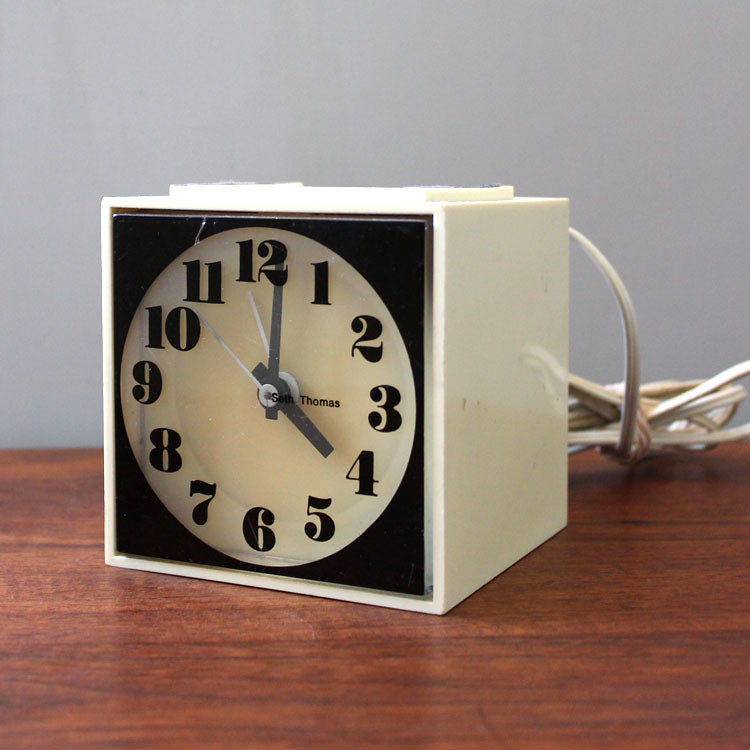This high-resolution photograph captures a vintage, 1970s-style square clock resting on an orangey-toned wooden table, with visible wood grain adding texture to the scene. The clock has an off-white face, adorned with black numerals and two black clock hands alongside a contrasting white second hand. Notably, part of the clock's covering is cracked, and the surface has visible scuff marks, suggesting its age and wear. A white cord protrudes from the back, slightly bunched and tangling towards one side. The backdrop features a plain white wall, creating a clean contrast with the clock and table. Prominently displayed on the clock's face in black font is the brand name "Seth Thomas."